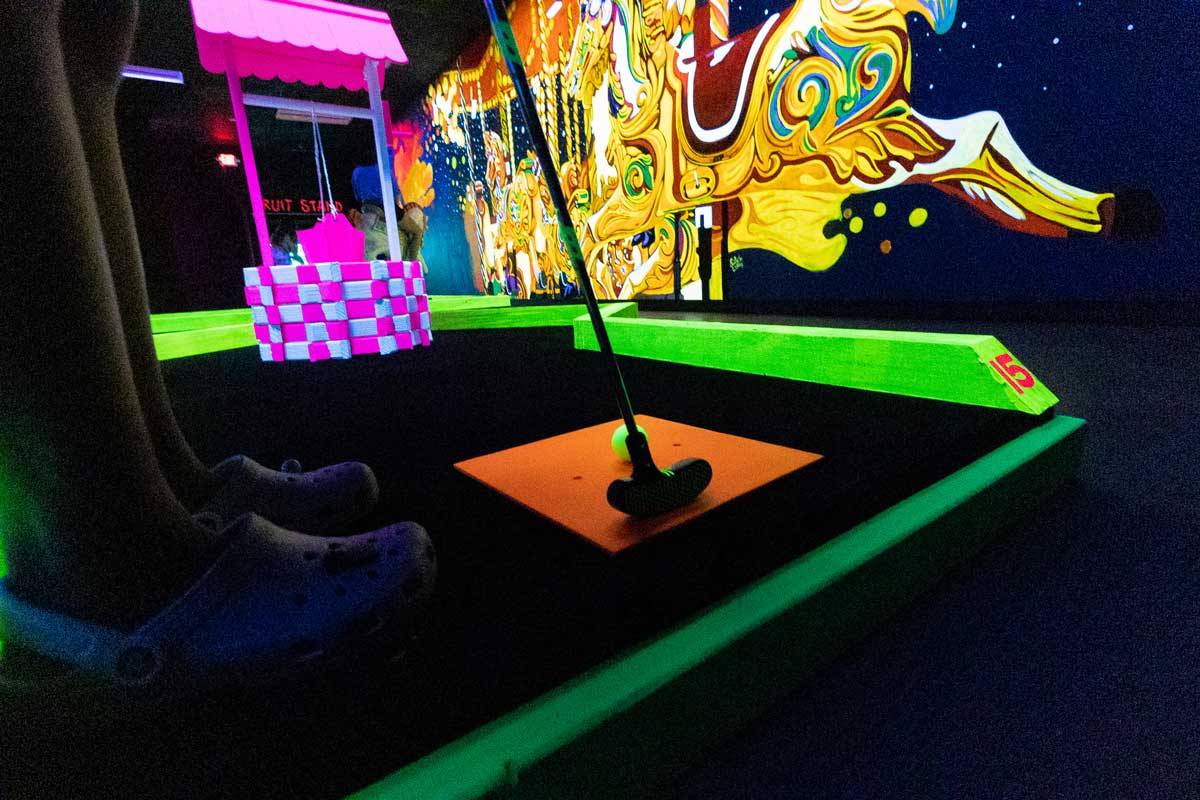The image captures an indoor miniature golf course, featuring a lively and vibrant scene under blacklight illumination. At the center is a person, likely a woman, wearing white Crocs and holding a putter. She is standing on an orange platform and is about to putt a fluorescent green golf ball. The scene is adorned with neon and bright colors, enhancing the playful atmosphere. In the middle of the course, there's a pink and white water well, serving as an obstacle on the hole. The hole itself is the 15th, marked by a green railing with the number 15. The backdrop includes a striking mural with yellow, blue, gold, and red hues, depicting what seems to be a carousel horse, adding to the whimsical nature of the environment. The overall setting suggests a fun, casual game designed with children in mind, filled with glowing fluorescent elements that stand out against the dark background.